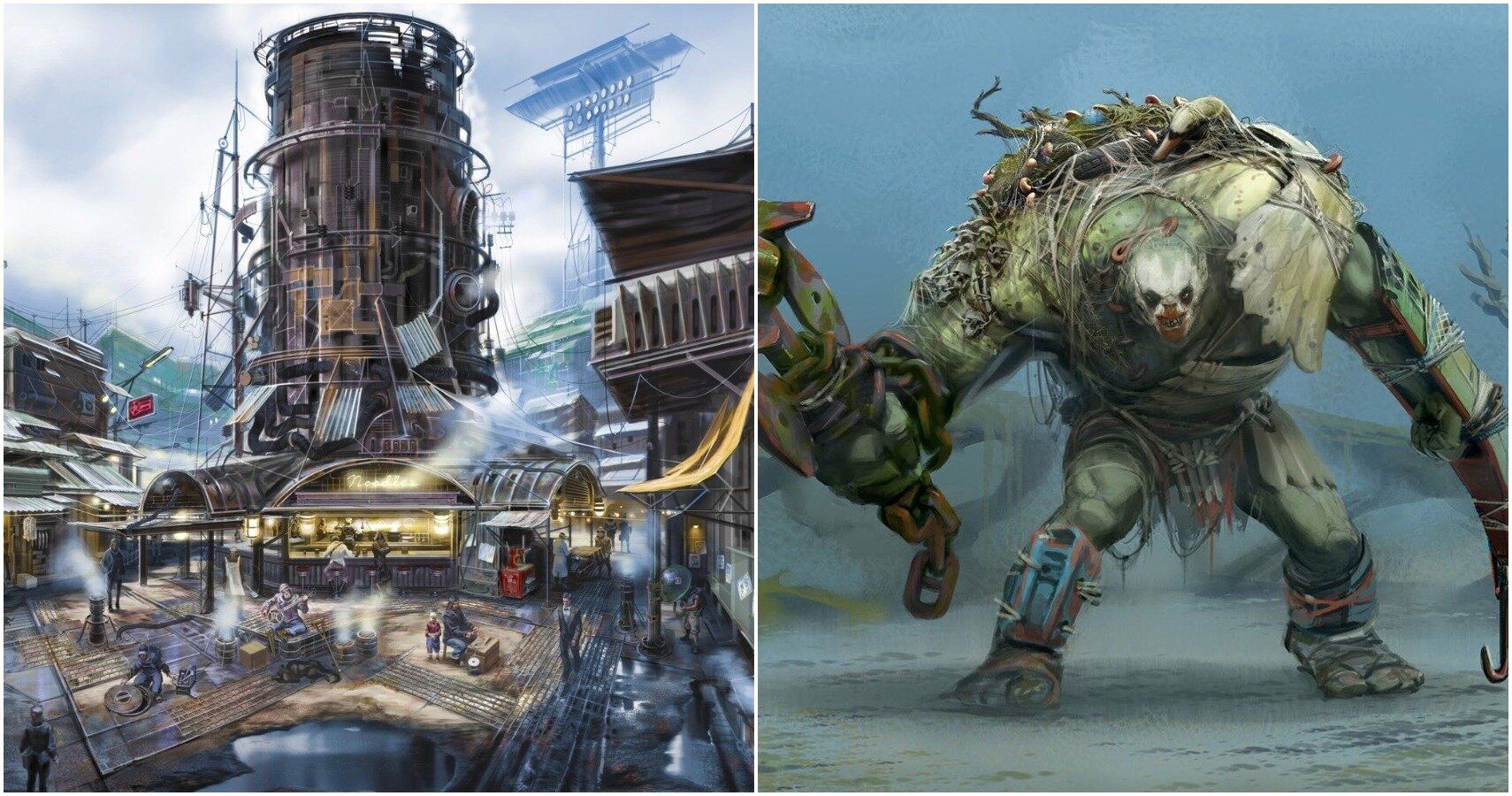The image appears to be a piece of detailed fantasy artwork, possibly concept art for a game or TV show rooted in an apocalyptic steampunk aesthetic reminiscent of Fallout 4. The left side of the image depicts a bustling market scene within Diamond City, characterized by a tall, precarious tower adorned with pipes, boards, and makeshift structures. At the base of the tower, various concession stores operate, including one notably labeled "Noodle Jewels," where several people are engaged in daily activities—some sitting at a bar, an older person and a child behind a box, a musician playing with an animal resting nearby, and others navigating the environment, such as an individual moving a manhole cover.

Dominating the right side of the artwork is a fearsome, hulking figure—a green-skinned super mutant. This imposing character carries a massive metal weapon and adorned its broad shoulders with skulls. With heavily-armored legs and an ambiguous hook-like object in its left hand, this super mutant adds an intense and menacing presence to the scene. The image, rich in details, combines elements of post-apocalyptic survival with fantastical, larger-than-life characters, effectively capturing the viewer's imagination.